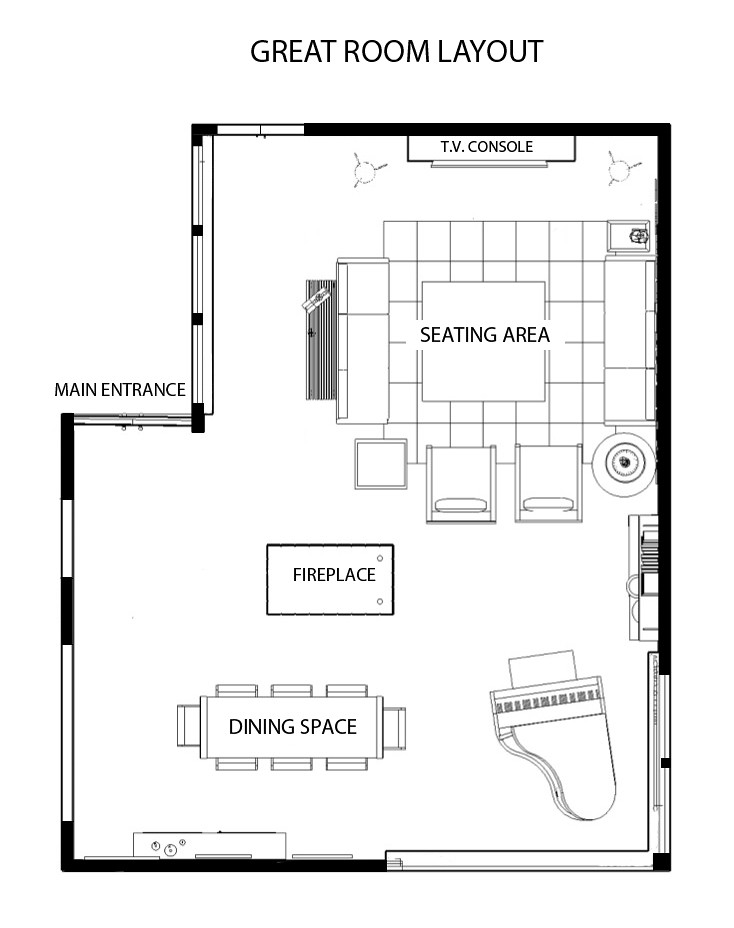This detailed black and white line drawing serves as a blueprint for a Great Room Layout in a house, depicted from a bird's-eye view. The room is predominantly rectangular, with a small rectangular section removed from the top left corner, which is labeled as the Main Entrance.

At the top right, there is a designated area for a TV Console. Moving downward towards the center of the drawing, a large Seating Area is illustrated, with a text box indicating its purpose. This seating configuration includes couches on the left and right sides, and two large chairs positioned at the bottom, all facing towards the TV Console area.

Central to the room, there is a labeled Fireplace, suggesting a prominent freestanding fixture. Below this central area, toward the bottom of the room, a Dining Space is outlined. This dining area features a rectangular table accompanied by six chairs along the top and bottom edges, and a chair on each side, emphasizing its capacity for hosting larger gatherings.

In the bottom right corner of the room, a grand piano is depicted, highlighting the room's multifunctional design that combines entertainment, relaxation, and dining in one cohesive space.